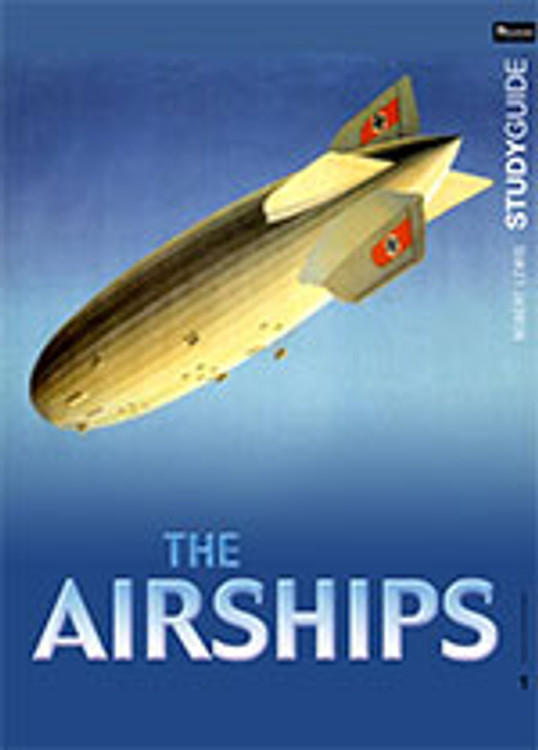The image depicts an airship, specifically resembling a blimp, in flight against a very dark blue and light blue background, giving the impression it's soaring through the sky. The blimp is painted in white, yellow, and black, with distinct designs on its wings or fins – red flags with black crosses flanked by white lapels. Its shape is broad at the front, narrowing and pointed at the back, akin to a cucumber with four rear fins. This airship is angled diagonally, head pointing downward to the left and tail upward to the right. Bold blue and light blue text at the bottom spells out "THE AIRSHIPS," while vertically aligned text on the right side of the image, in bold white and blue letters, reads "STUDY GUIDE," with some smaller, indistinct white text above it. Additionally, a rectangular logo in the top right corner features a black background with white text.